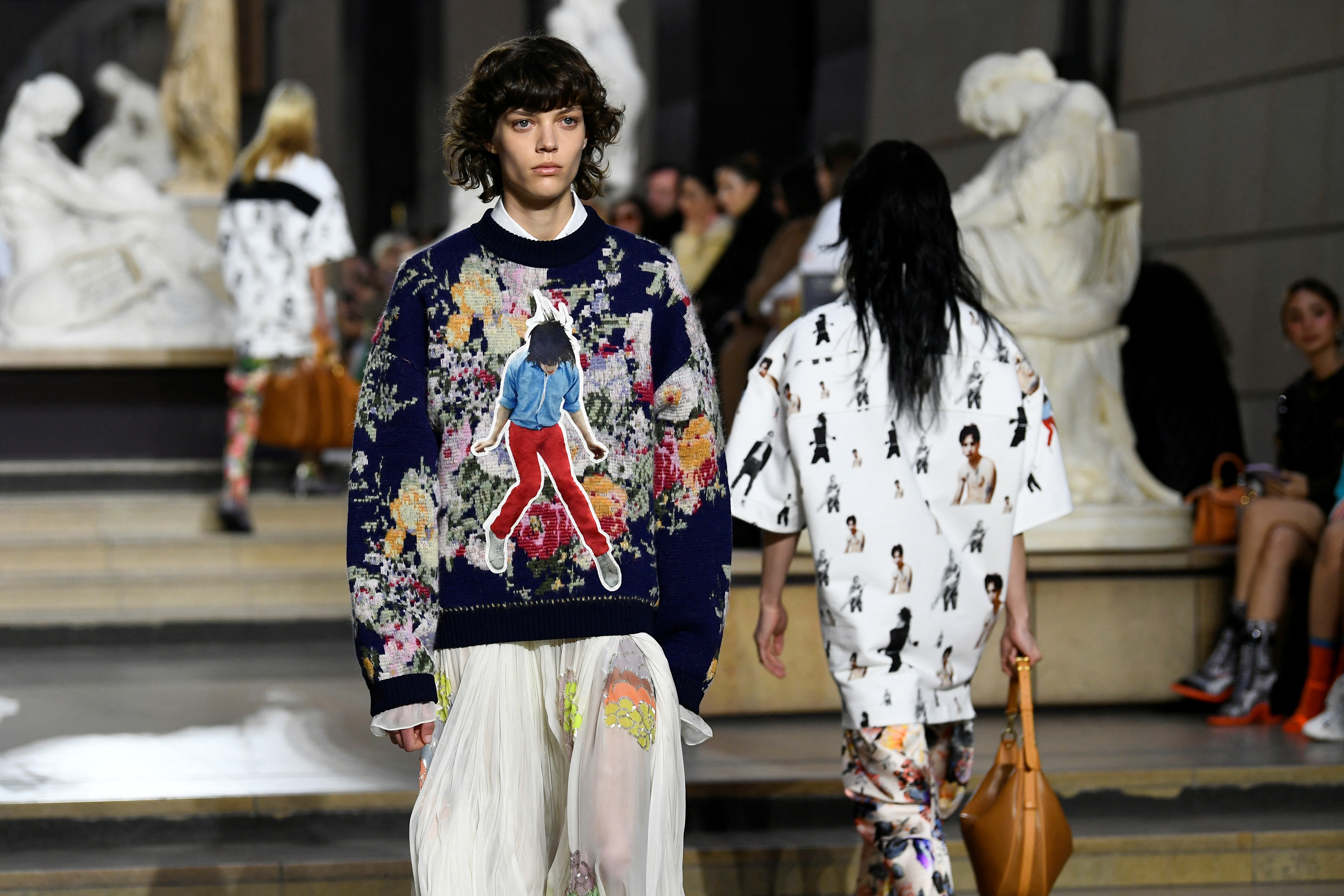The image captures a meticulously detailed fashion runway show set in what appears to be an art gallery, indicated by the marble statues and sculptures in the background. The photo is high-quality and taken indoors with a horizontal orientation. Two models dominate the scene: the closest one, a gender-neutral individual with sharp gaunt cheekbones and short black hair, strides towards the camera but is not looking directly at it. They wear a colorful, interesting sweater adorned with floral prints and a distinctive graphic of a dancing girl, which almost looks photoshopped onto the garment. Complementing the sweater are white pants. Behind this model, another person walks away; they have longer hair and sport a multicolored outfit that includes a white short sleeve shirt featuring images of people. Around the runway are numerous spectators, seated and keenly observing the show. The atmosphere, coupled with the striking and eclectic fashion, lends an air of professional elegance, further emphasized by the sharpness and clarity of the image.